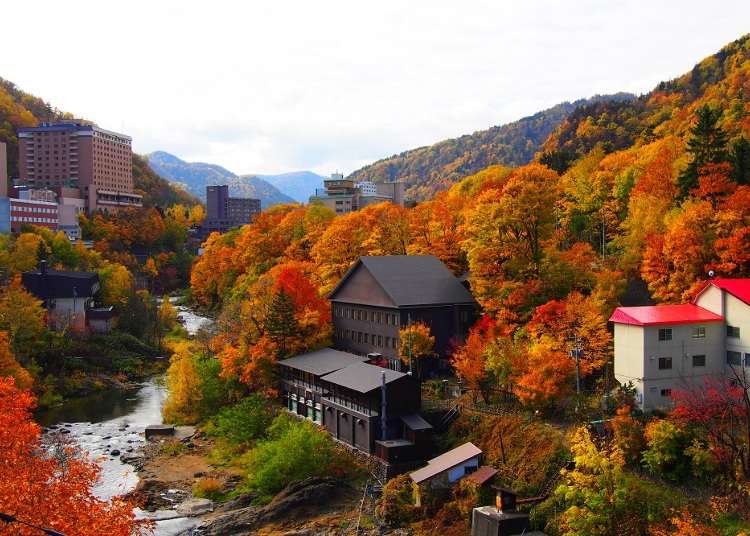This vibrant photograph captures a scenic autumn landscape of a rural town nestled among hills or mountains. The image prominently features a variety of buildings, including a dark wood-colored house with a black roof at the center, a white building with a red roof to the right, and several tall brick buildings on the left. A stream meanders through the middle of the town, bordered by numerous trees that are ablaze with autumn colors—shades of orange, red, yellow, and occasional patches of green. The town appears busy, with business-like structures, including a notable ten-story-high brick building. In the background, the majestic mountains stand tall, devoid of decorations, under a bright sky that transitions from a vivid white to a light blue hue.